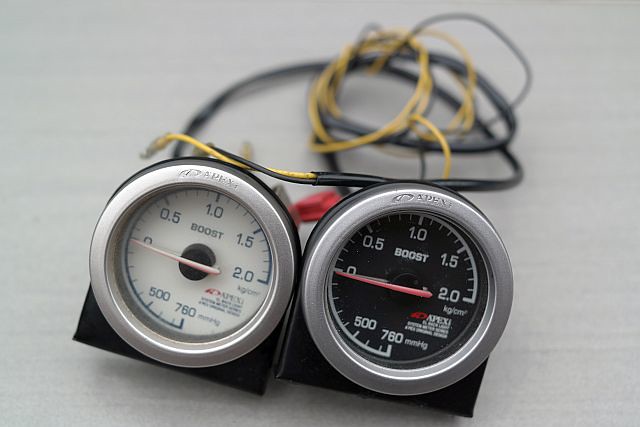On a gray background, two silver-rimmed gauges display their metrics with precision. The gauges are arranged side by side, with one featuring a white face and the other a black face. Each gauge ranges from 760 to 0 and then from 0 to 2.0, indicative of their measurement spectrum. The white-faced gauge is equipped with a silver hand, while the black-faced gauge boasts a striking pinkish-red hand. Both gauges are fitted with wires, one yellow and one black, which are encased in black plastic tubing that curls elegantly behind the devices. A small red component is situated beneath the gauges, adding contrast to the setup. These gauges are mounted on a black structure that folds underneath them, providing stability and support. Each gauge bears the word "Boost" on its face and is produced by the company Apex, highlighting their purpose and origin.